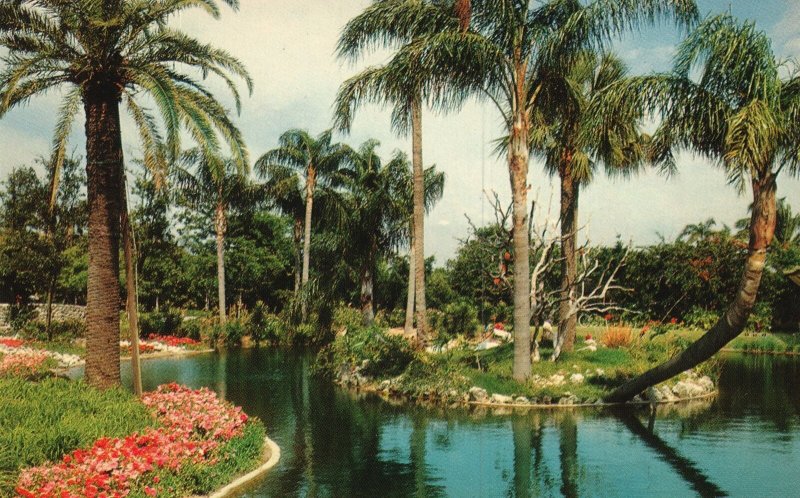This vintage colored photograph, marked with a few scratches and dust, captures a serene, well-manicured garden scene. Taken during the daytime under mostly clear blue skies with some large, puffy white clouds, the image radiates a tranquil atmosphere reminiscent of tropical destinations like Florida or Hawaii. At the center is a calm, clear pond with a small, grassy island that supports several palm trees, one of which arches gracefully over the water. The landscape is adorned with a variety of vibrant flowers: clusters of pink and white blooms on the left, and red flowers nestled under the trees. The garden is meticulously maintained, featuring both lush greenery and a dead tree that adds a natural touch to the composition. The overall peaceful ambiance and classical aesthetics evoke a sense of timeless beauty.